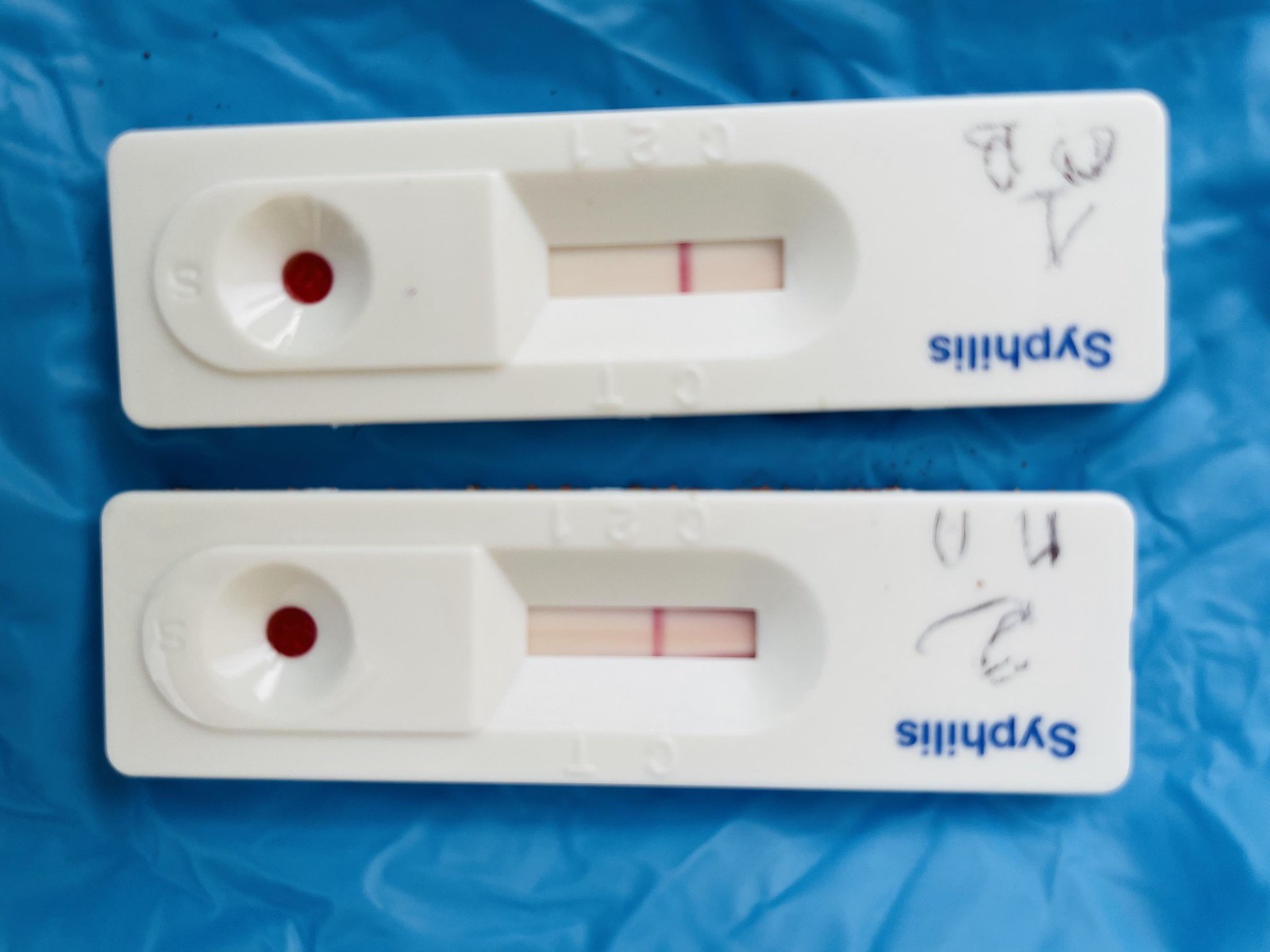In this photograph, two plastic testing devices, resembling pregnancy tests, are positioned side by side on a crumpled blue paper background. They appear to be syphilis test kits, as indicated by the label "SYPH" on each device. Both tests are upside down, with elongated, rectangular shapes common to similar diagnostic tests.

The central feature of each test is a hollow, bowl-like depression designed for liquid sample application. This area is filled with a dark red substance, presumably the test reagent. Each test strip contains a large stripe and is marked with a distinct set of initials, differing from one another. The tests bear a distinctive design, indicating regions that display results, typically positive or negative, based on the visual stripe pattern.

Overall, the image captures the clinical nature of these diagnostic tools, highlighting their functionality and purpose within a medical context.